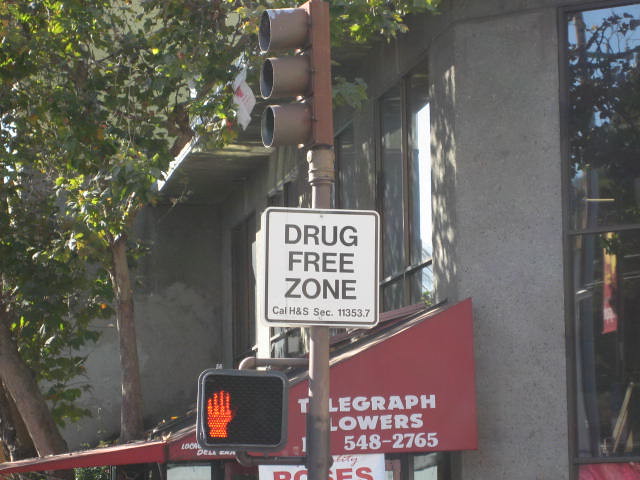The image depicts a city scene featuring a prominent "Drug-Free Zone" sign that references Cal H&S SEC 11353.7. This sign is mounted on a tall silver pole positioned centrally in the photograph. Below the main sign, there is a pedestrian signal, illuminated with the orange hand icon, indicating that pedestrians should wait due to incoming traffic. 

In the background, the setting appears to be in front of a gray building characterized by large, divided windows that line the facade. The structure includes a gray brick wall and a section that curves backward about two-thirds into the frame. On the left side of the image, partially obscured are two trees, their green foliage reaching up towards the building’s height.

Adding to the urban landscape, slightly right of the center and below the windows, is a red slanted awning adorned with white text reading “Telegraph Flowers,” accompanied by a phone number "548-2765." This awning extends off the picture’s right edge. The lighting indicates it is daytime, suggesting a bustling city environment, possibly hinting at New York.